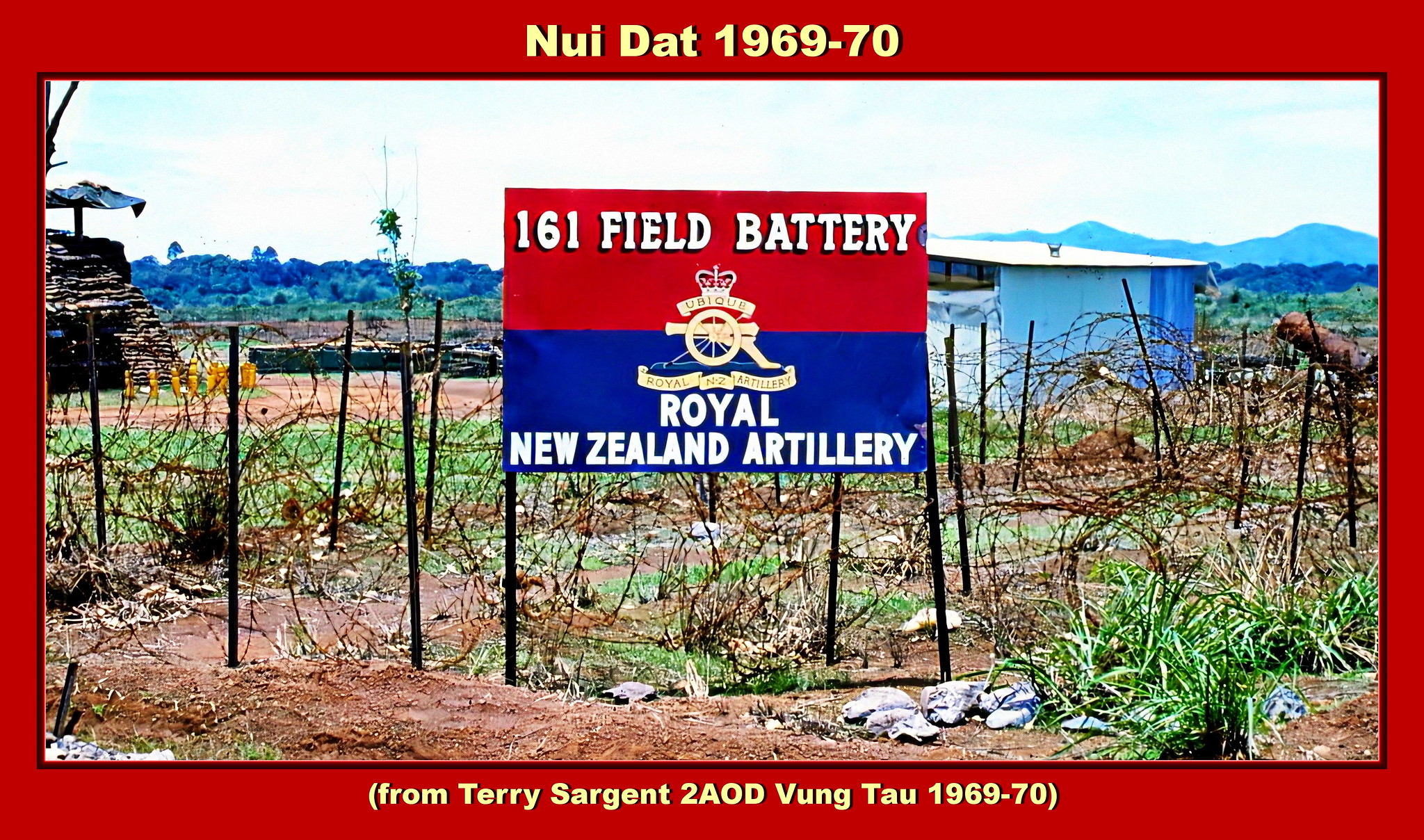The photograph, framed by a red border with yellow text above and below, displays a scene from Nui Dat, Vietnam, dated 1969-70. The top caption reads, "Nui Dat 1969-70," while the bottom states, "From Terry Sargent to AOD Vung Tau 1969-70." In the image, a large banner secured to the ground by poles prominently features the text "161 Field Battery Royal New Zealand Artillery," along with a logo resembling an old-style cannon, and a New Zealand flag. The banner itself is red on the top half and blue on the bottom half, with white lettering. The terrain is mostly barren, consisting of dirt, rocks, and patches of sparse grass, with rusty barbed wire fencing scattered about. To the left, a small stone structure with an umbrella is visible, while further back, on the right side of the banner, stands a white or light blue shed. In the distance, majestic mountains form the backdrop of the scene.